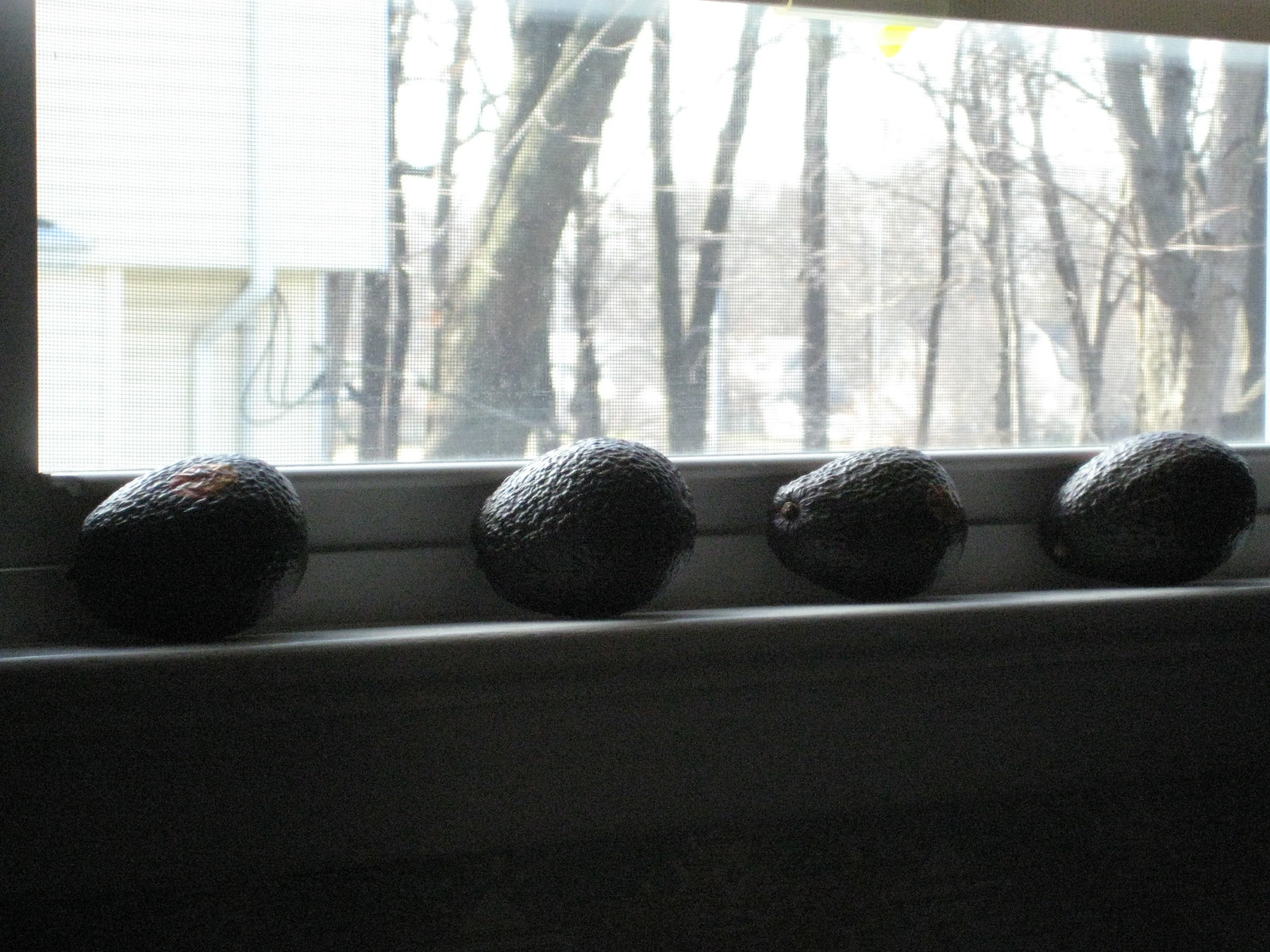In this image, four dark avocados are lined up horizontally on the edge of a wide, rectangular windowsill. Each avocado is placed on its side with the tip pointing leftwards. The windowsill itself is predominantly white with black accents. The indoor setting appears dimly lit, casting significant shadows. Through the window, the bright sunlight penetrates, illuminating the scene outside, which consists of a forest with numerous leafless trees and branches. The sky outside is a stark white or light gray, reflecting the abundance of sunlight. A white building can also be seen directly across from the window. This scene suggests it is someone's home, likely photographed in the early or late afternoon, with a forested backyard visible through the screened window.